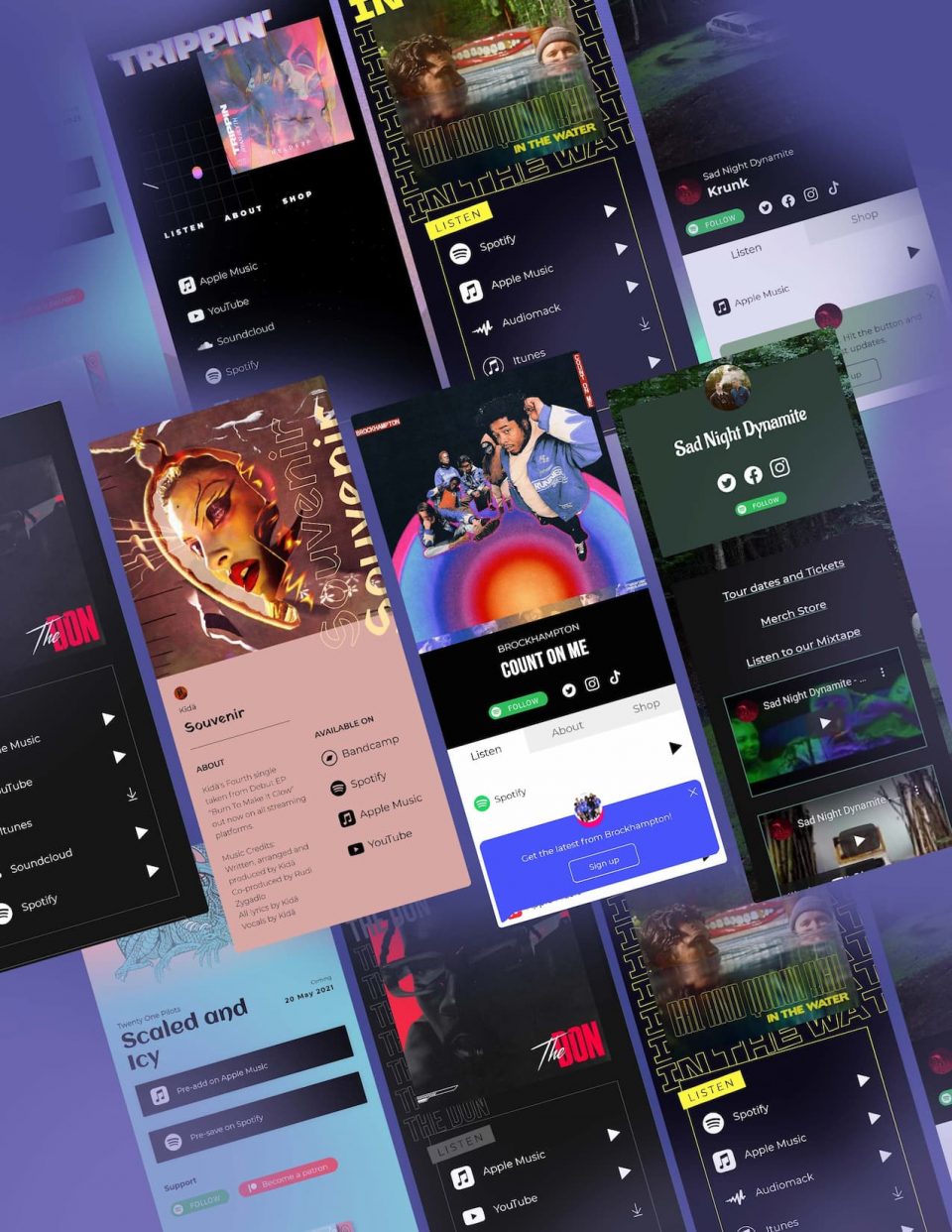The image depicts a collection of smartphone screenshots showcasing various album covers arranged in a visually engaging layout against a light purple background. 

Starting from the top, the featured album is "Trippin," characterized by its psychedelic design that evokes an acid trip vibe. Directly below and to the left of "Trippin" is the album "Souvenir," which displays an image of an Indian woman adorned with elaborate makeup. 

Next to "Souvenir" is "Count On Me" by Brockhampton, a cover featuring a group of Black men dressed in matching blue windbreakers and t-shirts. Following this is "Sad Night Dynamite," which, notably, does not have a discernible cover image.

At the bottom of the layout, there are three more albums: "Scaled and Icy," displaying a partially visible ice dragon; "The Don"; and "In The Water," which features two figures treading water. The light purple background of the setup visibly masks additional music options, adding a layer of intrigue to the arrangement.